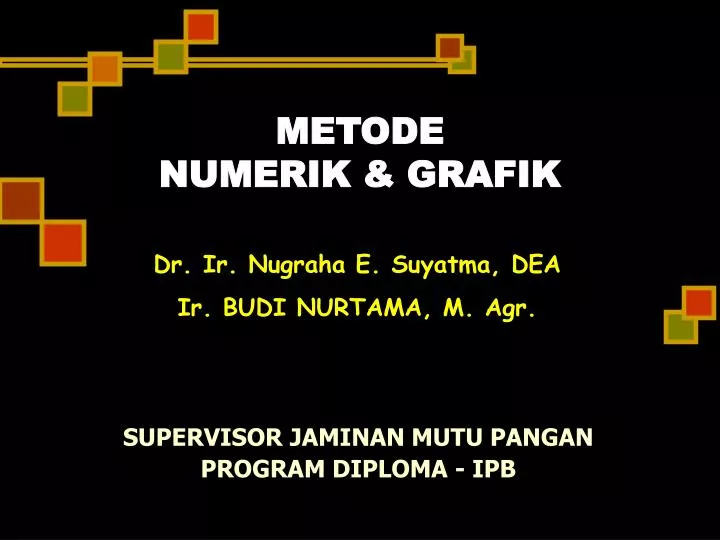The image features a black background with multiple colored elements, including squares filled with red, green, orange, dark brown, and yellow lines dividing sections of the image. At the top center, in large white text, it reads "METODE, NUMERIC, AND GRAPHIC." Directly below, in yellow text, are the names and titles "DR. IR. NUGRAHA E. SUYATMA, DEA." and "IR. BUDI NURTAMA M.AGR." Further down in white text, it states "SUPERVISOR JAMINAN MUTU PANGAN, PROGRAM DIPLOMA IPB." The top left corner of the image is marked by a black line that stops halfway and is bordered by blocks filled with the same array of colors, enhancing the structured yet vibrant design of the image.